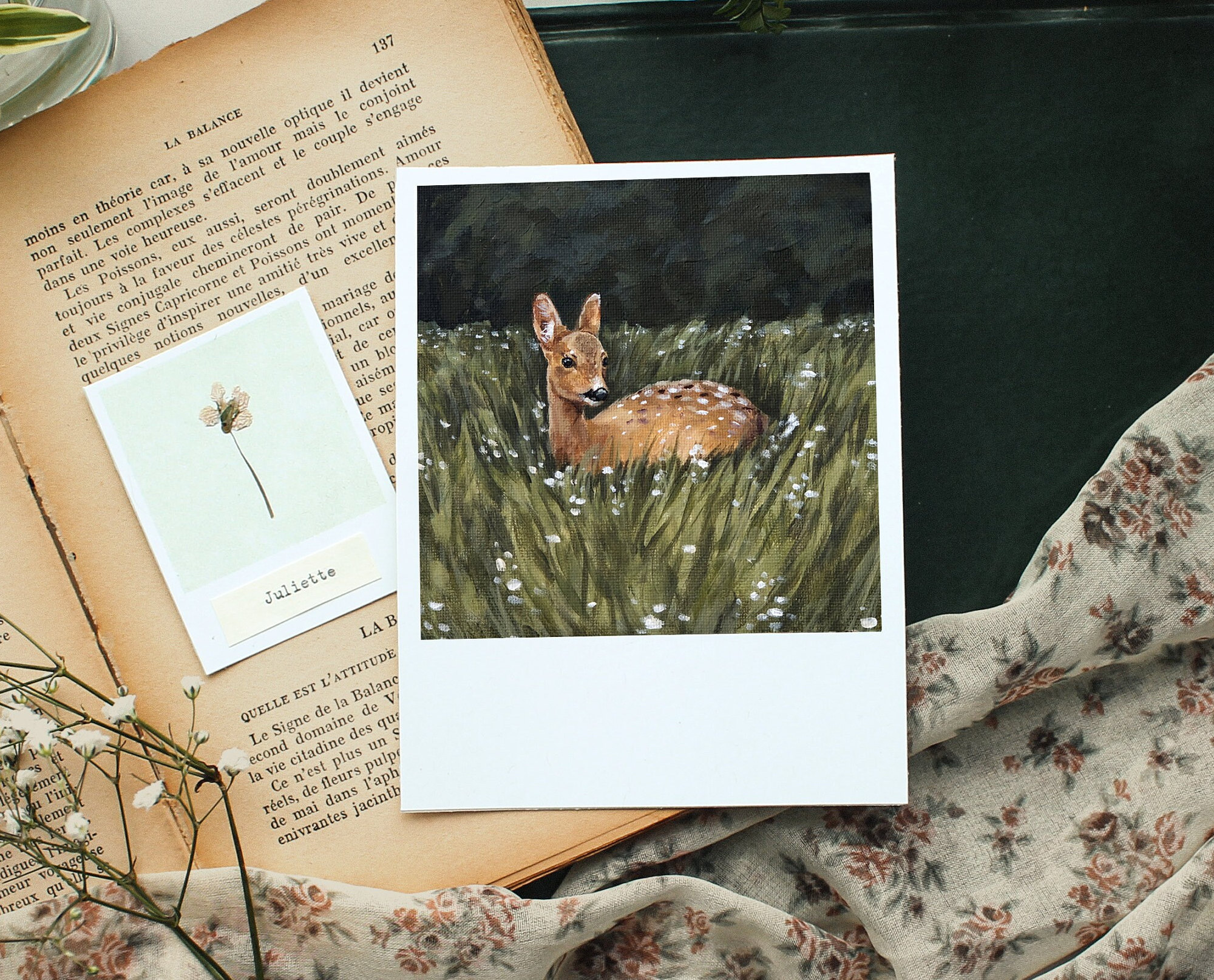The image depicts an artfully arranged layout against a dark green background. At the bottom edge, a linen sheet with a delicate floral pattern frames the scene. In the lower left corner, partially resting on the sheet, lies a small green branch adorned with tiny white flowers. Centered prominently is a white rectangular piece of paper, upon which a square photo is attached. The photo, housed in a Polaroid-style white frame, showcases a beautifully detailed drawing of a brown deer with white spots, nestled serenely in a meadow of tall green grass and white flowers.

This white piece of paper with the deer illustration is placed diagonally atop an open book, which appears notably aged, with its pages exhibiting a brownish hue. The book's visible spread includes the title "Law of Balance" and the page number 137. Written in French, the text is accompanied by a smaller sketch of a flower captioned "Juliet" on a beige segment stuck onto the page, partially obscuring the book's formal text.

Spread around the main focus, which is the photo and the book, the floral fabric curves around the bottom and up toward the right side of the image. Further enhancing the composition, additional white flowers are scattered around the bottom left, and there are traces of some sort of glass bowl with greenery peeking from the top left corner. The overall assembly presents a harmonious blend of artistic elements and natural beauty.